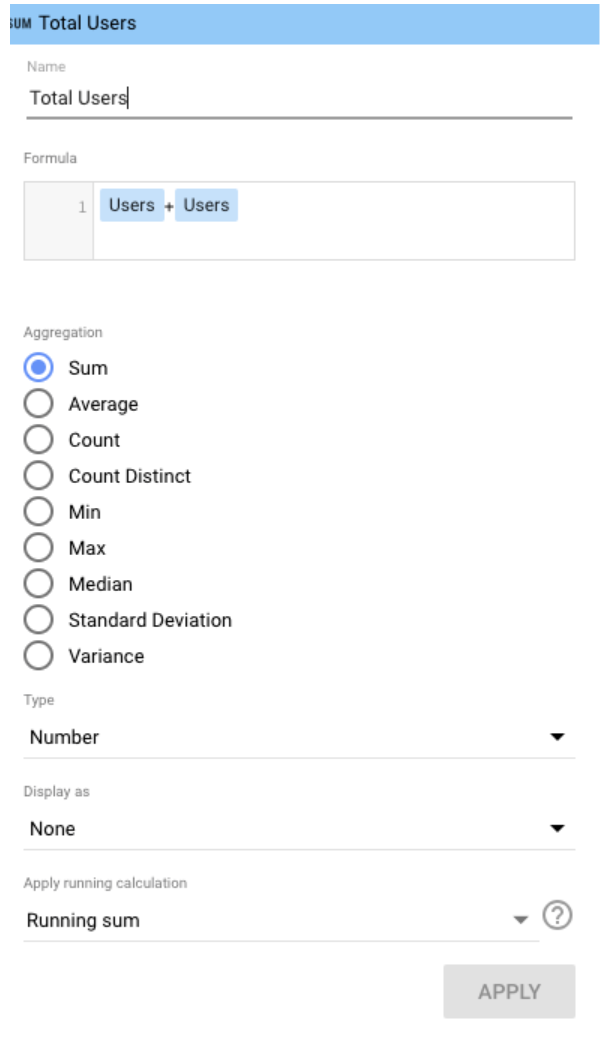The image showcases a form designed for statistical computations. At the top, there is a header labeled "Total Users," with a text box underneath it containing the typed words "Total Users." Beneath this is another section titled "Formula," featuring a text box that reads "users + users." Further down, under the heading "Aggregation," there is a variety of calculation options to choose from. These options include sum, average, count, count distinct, minimum, maximum, median, standard deviation, and variance, each accompanied by a corresponding button.

The form appears to be part of a statistical package or calculator, allowing users to perform various statistical techniques. Additionally, there is a drop-down menu labeled "Type," which includes the option "number," and another drop-down labeled "Display As," with "None" selected. There is also a checkbox for "Apply Running Calculation," and the option "Running Sum" is selected. Finally, at the bottom of the form, there is a greyed-out "Apply" button.